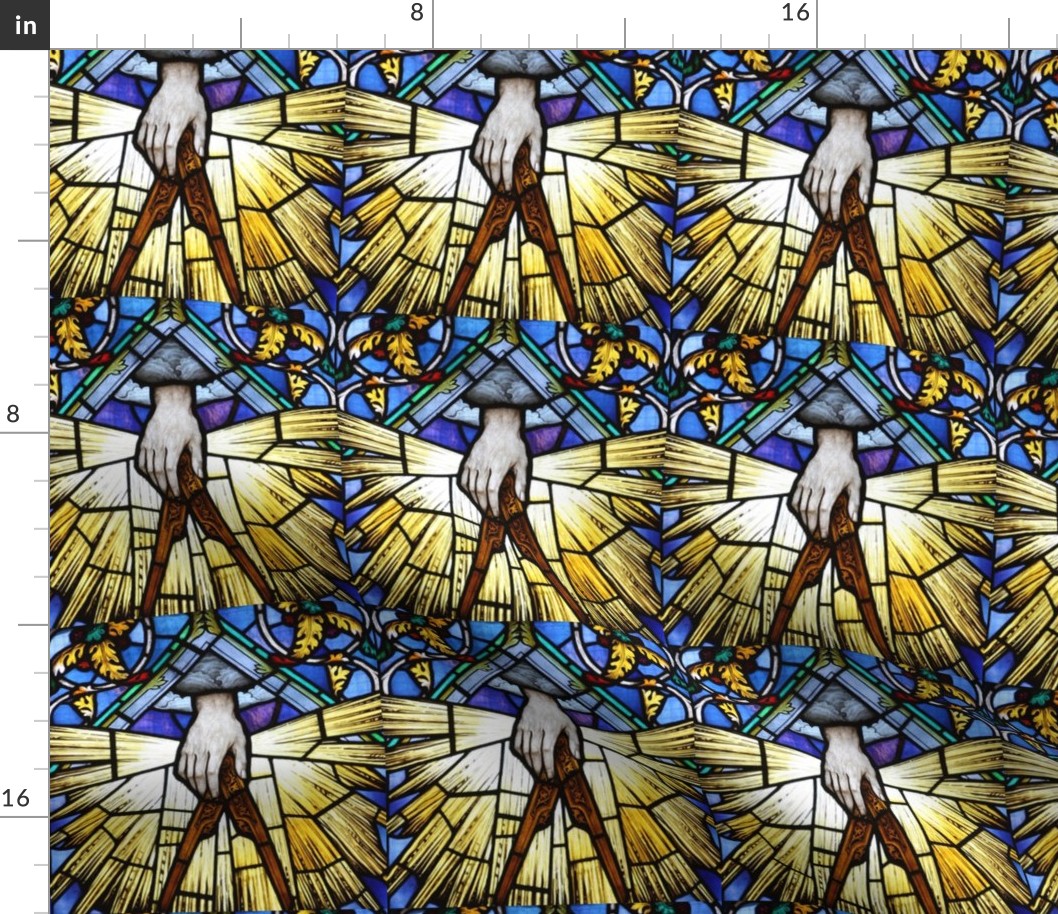The image showcases a repeated pattern resembling stained glass, forming a grid of nine visible sections arranged in three rows and three columns. Each section features a hand descending from the top, grasping what appear to be two wooden slabs. Radiant yellow light emanates from behind these slabs, creating an ethereal effect. Above and around the hand, intricate stained glass designs in rich hues of blue and purple are present, as well as golden leaves adorning the top left and right corners. A key detail in the image is a black square located in the upper left corner, containing the white letters "IN" along with incremental measurement lines, similar to those found on a ruler, labeled at intervals of 8 and 16 inches. This pattern is consistent across the grid, though some parts of the designs on the right side are partially cropped out.